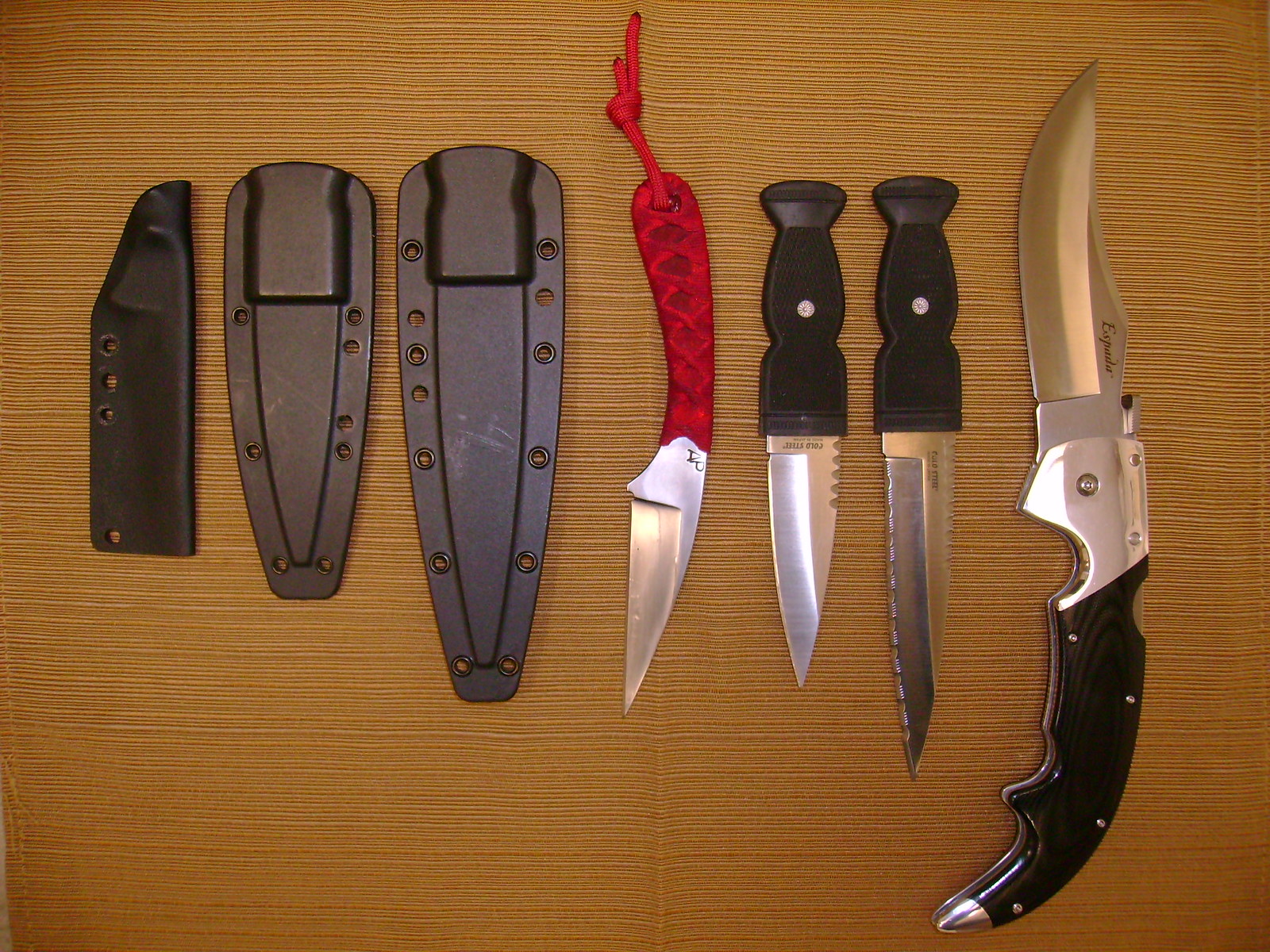The image features a detailed knife collection displayed on a light brown, canvas-like surface, possibly a table. On the left side of the image are three knife sheaths. The smallest one is a black holster with a flat backside and bottom, tapering slightly toward the top right. Next to it, there is a slightly longer sheath that also features a series of holes—three on the left, four on the right. The third sheath is very similar but slightly bigger. 

Moving to the right side of the image, there are four knives arranged from left to right. The first knife has a unique red handle with a dark pattern and a short, silver blade with the sharp edge facing left. A piece of fabric or lace extends from the handle, which looks like velvet or velour. To the right of this knife are two black-handled knives with identical pyramid-textured grips. The first black-handled knife has a serrated edge on the right and a sharp edge on the left, while the second has a longer blade with an extended serrated edge. Finally, on the far right is the largest knife, oriented vertically, with a long black handle adorned with four small silver dots. The handle's tip and top are silver, and the blade itself has a slight curve, with the sharp edge on the left and tapering into a point at the top.

Overall, this arrangement showcases the variety in the collection, with each knife having distinct features and corresponding protective sheaths.